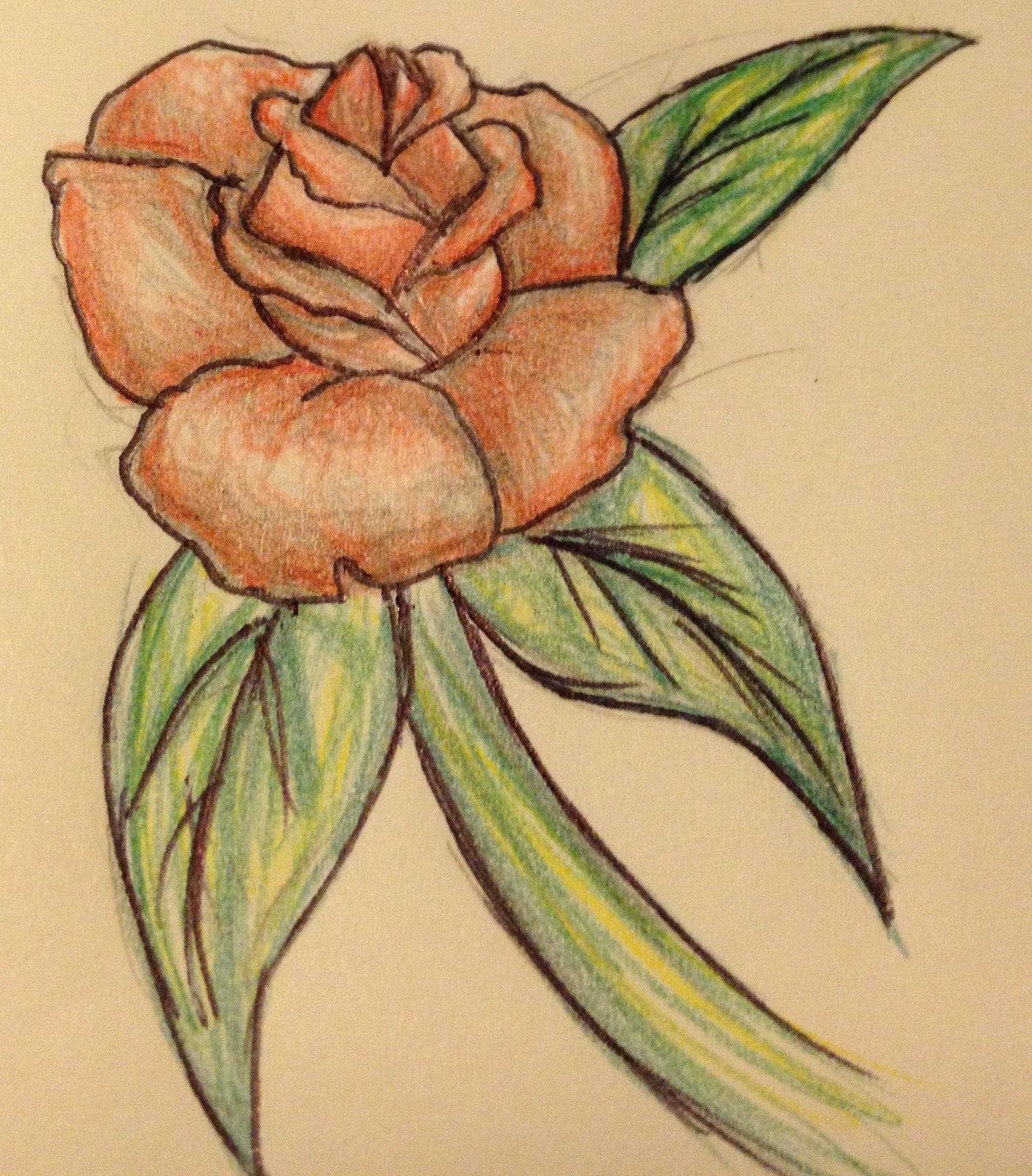This is a colored pencil drawing of a vibrant red rose, done on slightly off-white, light brownish paper. The rose is fully in bloom, featuring petals that are initially bunched up in the middle and gradually spread out towards the edges. The petals are red with subtle patches of white and outlined in black pencil, showcasing some prominent details, including larger, rolled-up inner petals and five larger outer petals. Surrounding the rose, there are three green leaves with a faint hint of blue around the edges and tips, as well as occasional streaks of yellow. One leaf points out from the top right, another from the bottom right, and the third from the bottom left. These leaves exhibit detailed black veins, with one main vein running down the center and smaller veins branching off. The green stem, which has traces of blue and yellow, curves gracefully from the base of the flower to the bottom right of the drawing. Some light, residual pencil sketches are visible around the leaves and flower, contributing to the overall artistic charm of the piece.